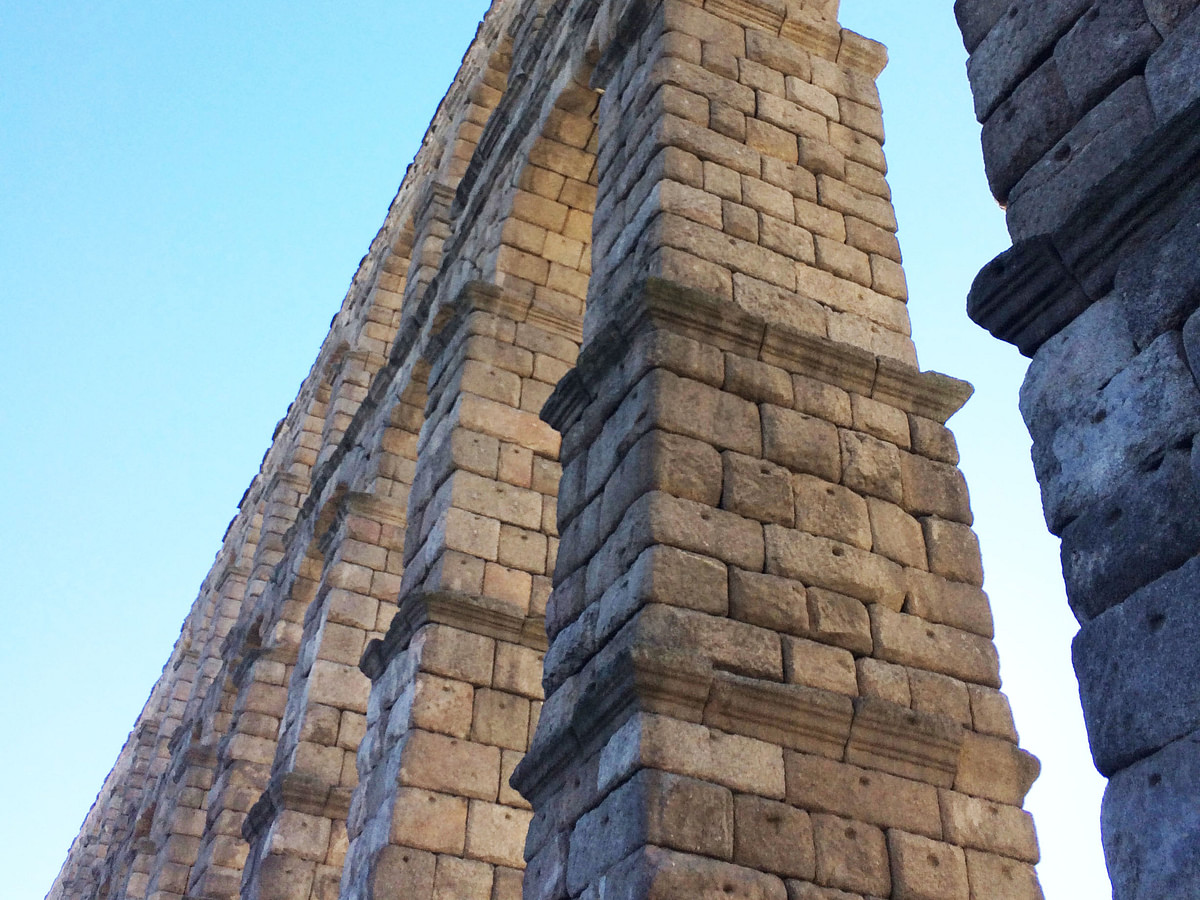The color photograph captures a portion of a tall, ancient stone structure with ornate columns, stacked using square rectangular blocks in various shades of browns and light tans. The picture is taken from the base, looking directly up, emphasizing the towering pillars that might lead to archways, although the angle only reveals their sides. In the bright, clear blue sky behind the structure, there are no visible animals, humans, machinery, or any inscriptions that might hint at the location, suggesting it might be historic and likely outside the United States. To the right, part of another structure is visible, made of darker stone, contributing to the overall mood of enduring antiquity.